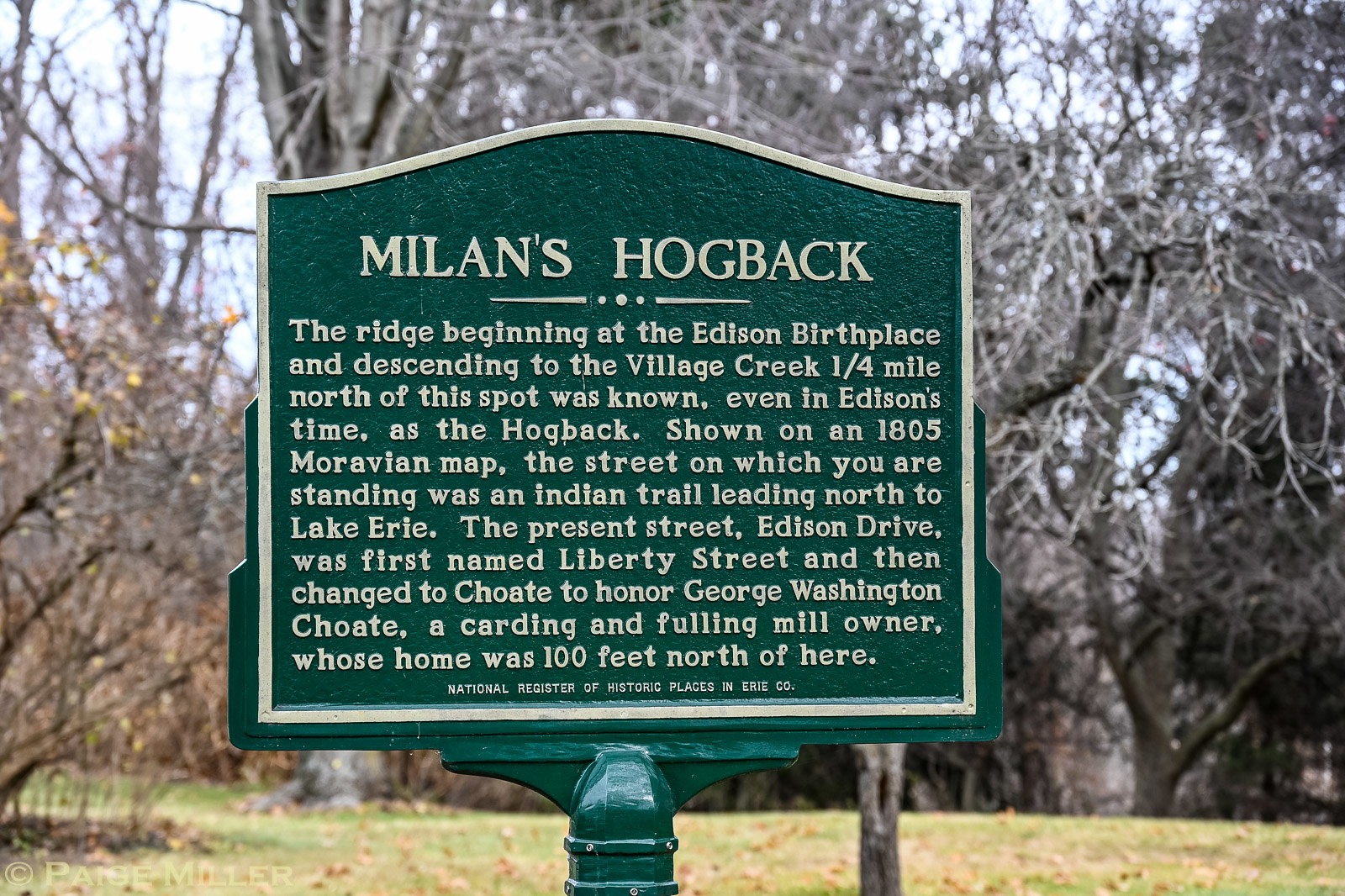This is a horizontally aligned rectangular image taken outside in a park-like setting within Erie County, Colorado. The focal point is a green metal sign with a curved top and a gray border, prominently featuring the title "Milan's Hogback" in large, all-caps light gray letters. The sign details the historic significance of the location, stating: "The ridge beginning at the Edison birthplace and descending to the Village Creek, a quarter mile north of this spot, was known, even in Edison's time, as the Hogback. Shown on an 1805 Moravian map, the street on which you are standing was an Indian trail leading north to Lake Erie. The present street, Edison Drive, was first named Liberty Street and then changed to Choate to honor George Washington Choate, a carting and foaling mill owner whose home was 100 feet north of here." At the bottom, in smaller all-caps text, the sign reads "National Register of Historic Places in Erie County." The background features a blurry view of a grassy lawn scattered with leaves, several tall, bare trees, a few of which have yellow leaves, and a visible blue sky with possible white clouds.